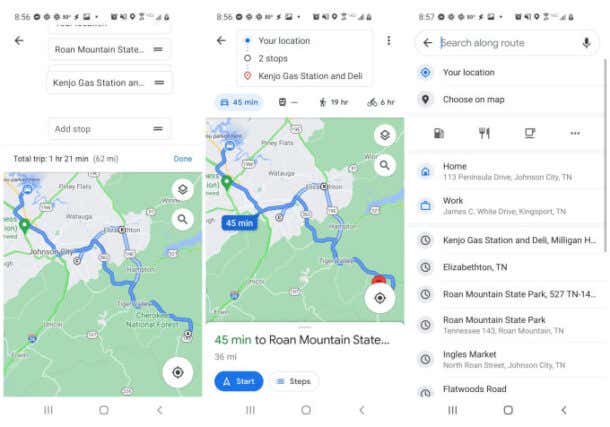This image showcases three screenshots of a cell phone, presumably displaying a navigation or map application, likely Google Maps. Each screenshot offers a different view of the app's interface, indicating a step-by-step progression through its features.

In the first image, the top of the screen displays status icons including the time (8:56), wireless signal strength, and battery level, confirming that it is a mobile device. The page is primarily white with black text. Here, we see a map with blue route markings and a label indicating "Total trip: 1 hour 21 minutes." The map also shows key destinations such as "Roan Mountain State Park" and "Kenjo Gas Station."

The second image continues from the first, showing a similar map view, but with updated information. At the top, it reads "Your location," followed by "2 stops." Specific stops include "Kenjo Gas Station" and "Delhi." The route is highlighted in blue, indicating "45 minutes to the destination" and "40 minutes to Roan Mountain State Park."

In the final image, a search box appears at the top where the user has typed in "Your location, choose on map." Below, it lists frequent locations such as "Home," "Work," and previously searched or suggested places like "Kenjo Gas Station," "Elizabeth, Tennessee," and "Roan Mountain." The three standard navigation icons typical of an Android device are visible at the bottom of each page, suggesting the use of an Android operating system.

This detailed series of images illustrates the functionalities of a navigation app, displaying routes, travel times, and location searches.